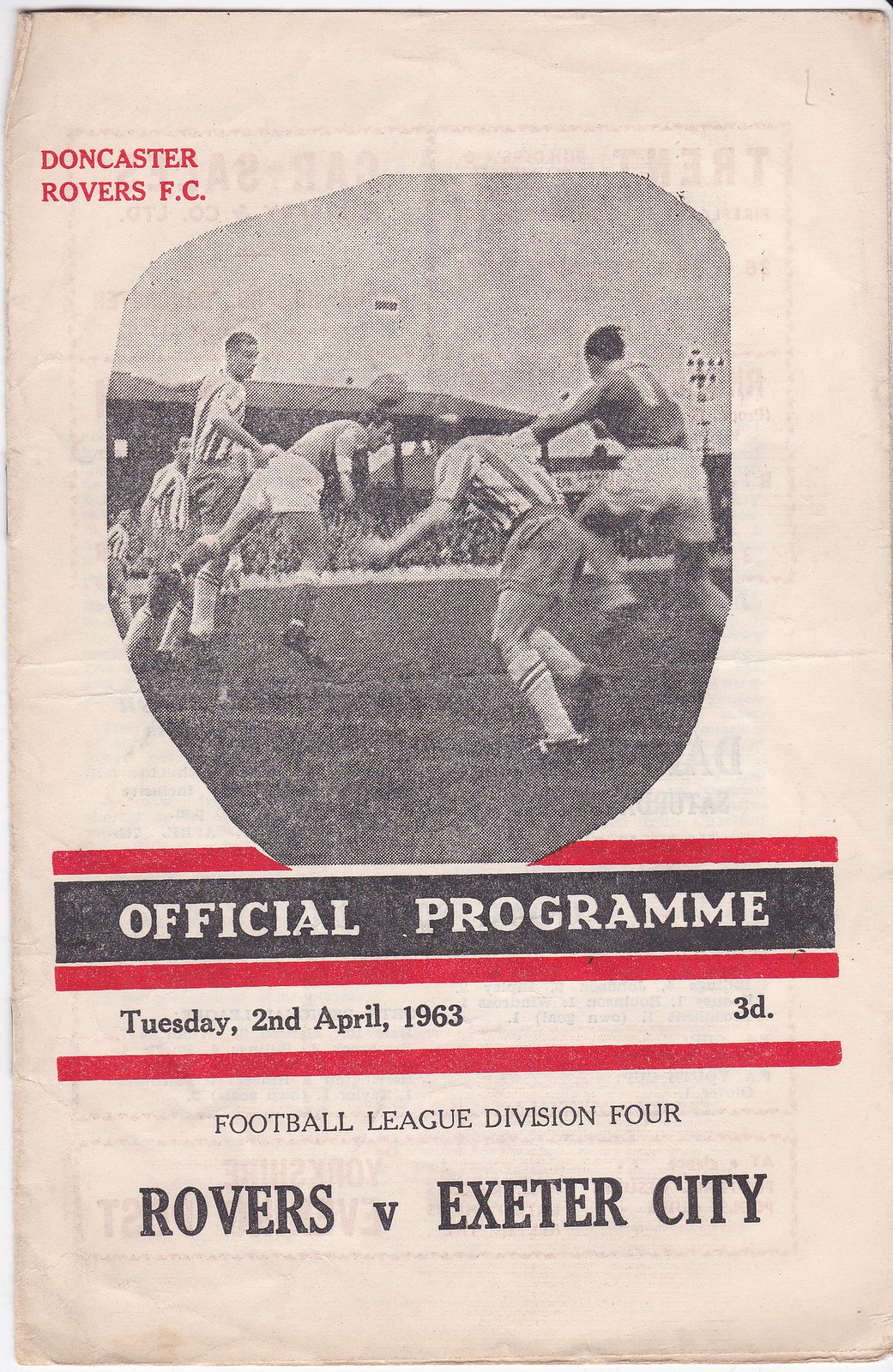The image features the aged cover of a soccer program from Tuesday, 2nd of April, 1963, now boasting a cream-beige background. At the upper left, it reads "Doncaster Rovers FC" in small red font. Dominating the center is an oval-shaped, black-and-white photograph capturing an intense moment in a soccer match, with four players prominently in action—two poised to head the ball, flanked by two others jumping on either side, and additional players and a crowded stand visible in the background. Below the photo, "Official Program" is emblazoned in large white letters against a black backdrop, adorned with thin red horizontal lines above and below. The details continue with the date, "Tuesday, 2nd of April, 1963" followed by the price "3D," both set against the cream background, punctuated once more by a red line. At the bottom, "Football League Division IV" is noted in smaller text, culminating in bold black letters announcing the match-up: "Rovers vs. Exeter City." The cover shows signs of age with slight crinkles and wrinkles along its edges.